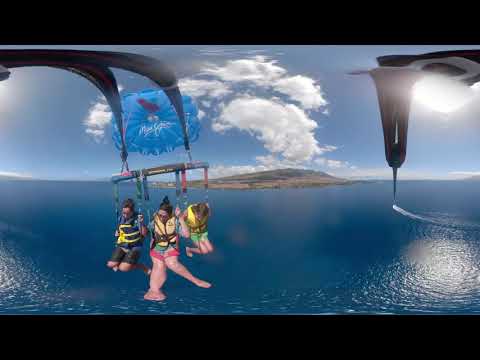The image depicts a detailed, wide-angle view of a family parasailing above a sparkling ocean on a sunny day with scattered clouds. The scene centers on a woman and two children, all wearing yellow life jackets, suspended from a sturdy lifting device with two long poles and hooks attached to handles. They are securely fastened and appear mid-air, possibly either ascending from or descending towards the water, their feet lifted. Behind them billows a large blue parachute with some written words on it, trailing in the wind. Below, the ocean glistens with sunlight, reflecting a bright white spot. In the background, a small island is visible beneath a partly cloudy blue sky. On the left side of the image, another empty lifting device mirrors the setup, emphasizing the expansive, carefree atmosphere of the adventure.